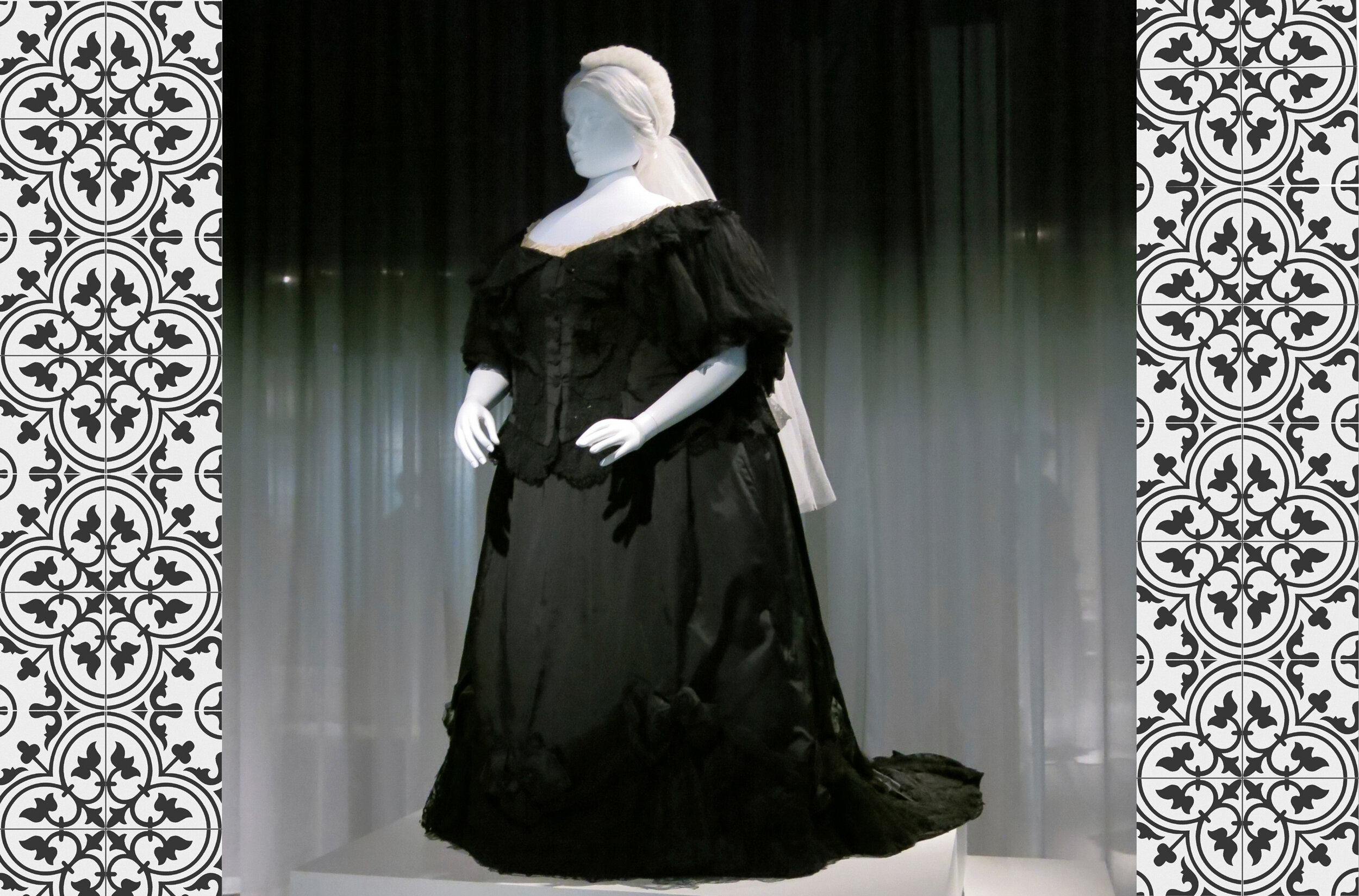In this photograph, a white mannequin with a heavier set figure is adorned in an elegant, long black gown, reminiscent of a wedding dress. The dress features ruffled shoulders that elegantly expose the mannequin's shoulders and has poofy, ruffled sleeves. The voluminous skirt drapes down beyond the legs, pooling onto the floor. The mannequin, standing on a white platform, has long, flowing white hair or a white headdress. A sheer gray curtain serves as the backdrop, with a spotlight highlighting the mannequin's presence. Framing the image on either side are decorative borders with black and white repeated patterns, adding a touch of intricate detail to the scene.